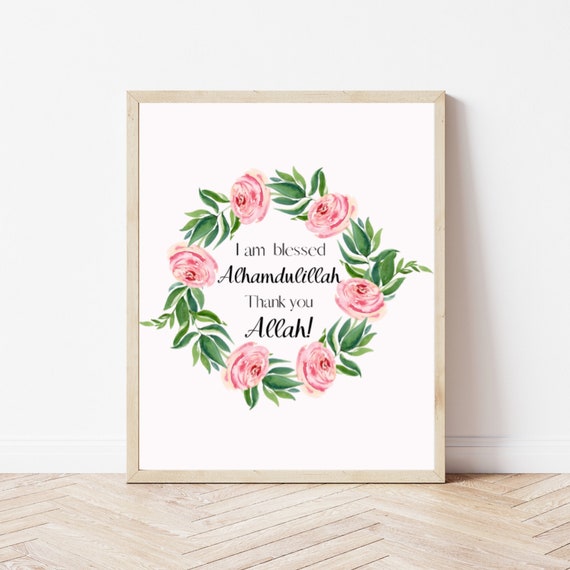The image depicts a framed photograph leaning against a white wall in what appears to be an indoor setting, possibly a living room. The floor consists of light tan, blonde floorboards that form a triangular arrow pattern. The frame itself is a light-colored wood, blending seamlessly with the floorboards. Inside the frame, against a white background, is a meticulously arranged wreath made up of green leaves and six pink rose-like flowers, forming a perfect circle. In the center of the wreath, black text reads: "I am blessed" at the top, followed by "Alhamdulillah" in script, "thank you" in print, and finally, "Allah!" with an exclamation mark at the bottom. There's a subtle shadow falling to the right side of the frame, suggesting a light source from the left.